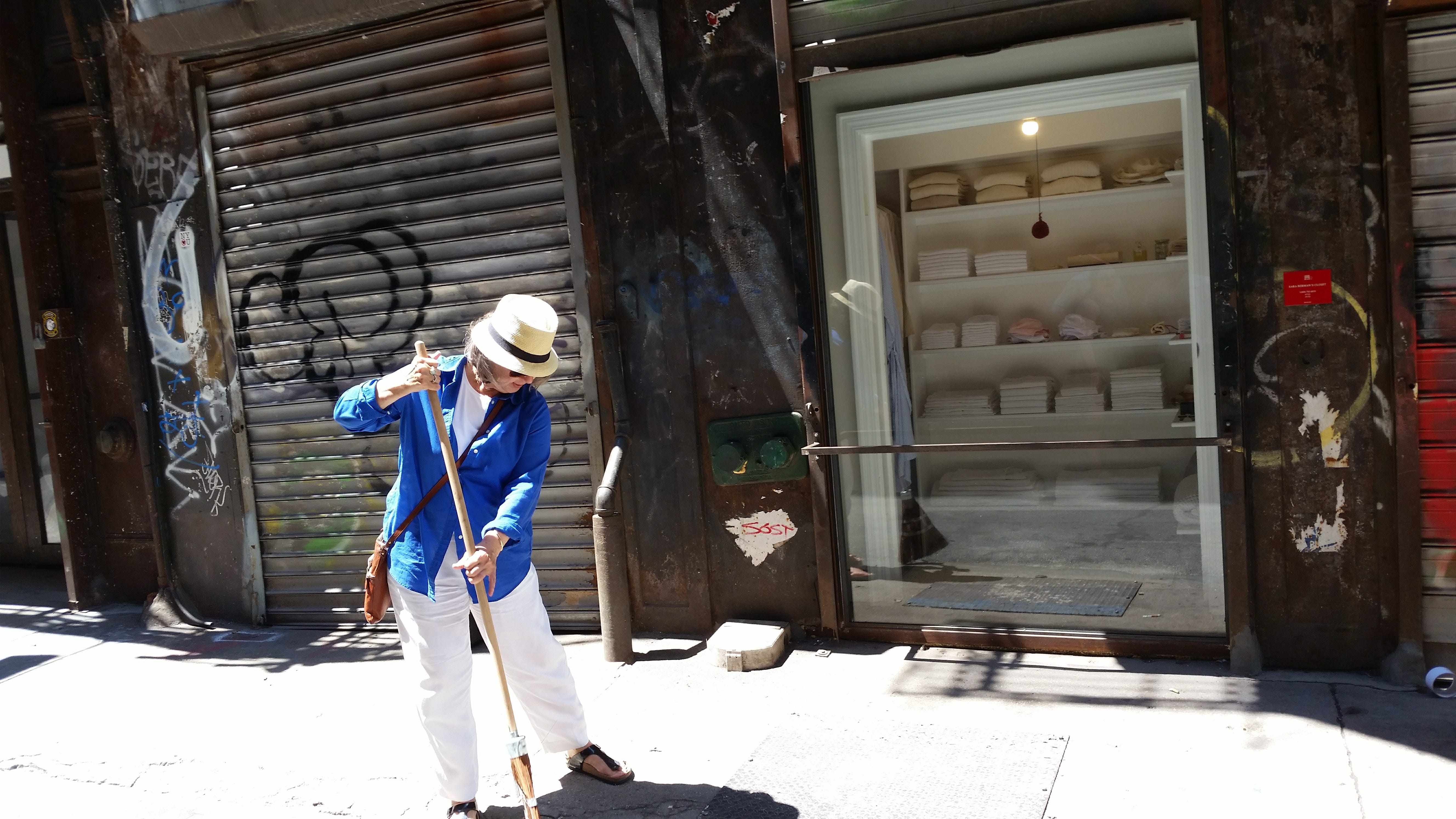In this image, a woman is sweeping a sunlit sidewalk in front of a dilapidated, graffiti-covered building that appears to be abandoned. The woman wears a striking outfit consisting of a blue, long-sleeved shirt, long white pants, black sandals, and a straw hat adorned with a black ribbon. A thin, square-shaped brown crossbody bag rests over her left shoulder. She is engaged in a sweeping motion, her right arm bent at the top of the broom and her left arm extended toward the middle. 

The background reveals more details of the rundown area, with rusty metal trim and an old, silver garage door defaced by black spray-painted graffiti. The structure has multiple garage doors, skinny and shabby, with a dark brown and rust-colored steel beam to the right. There is also a glass front door with white trim, unexpectedly clean and modern in contrast to its surroundings, showing neatly arranged towels on a four-tier rack inside, visible through the glass. A metal bar covers the glass door for added security. The sunlit concrete sidewalk she is cleaning has bright patches from the sun, further emphasizing the stark environment she's tending to.